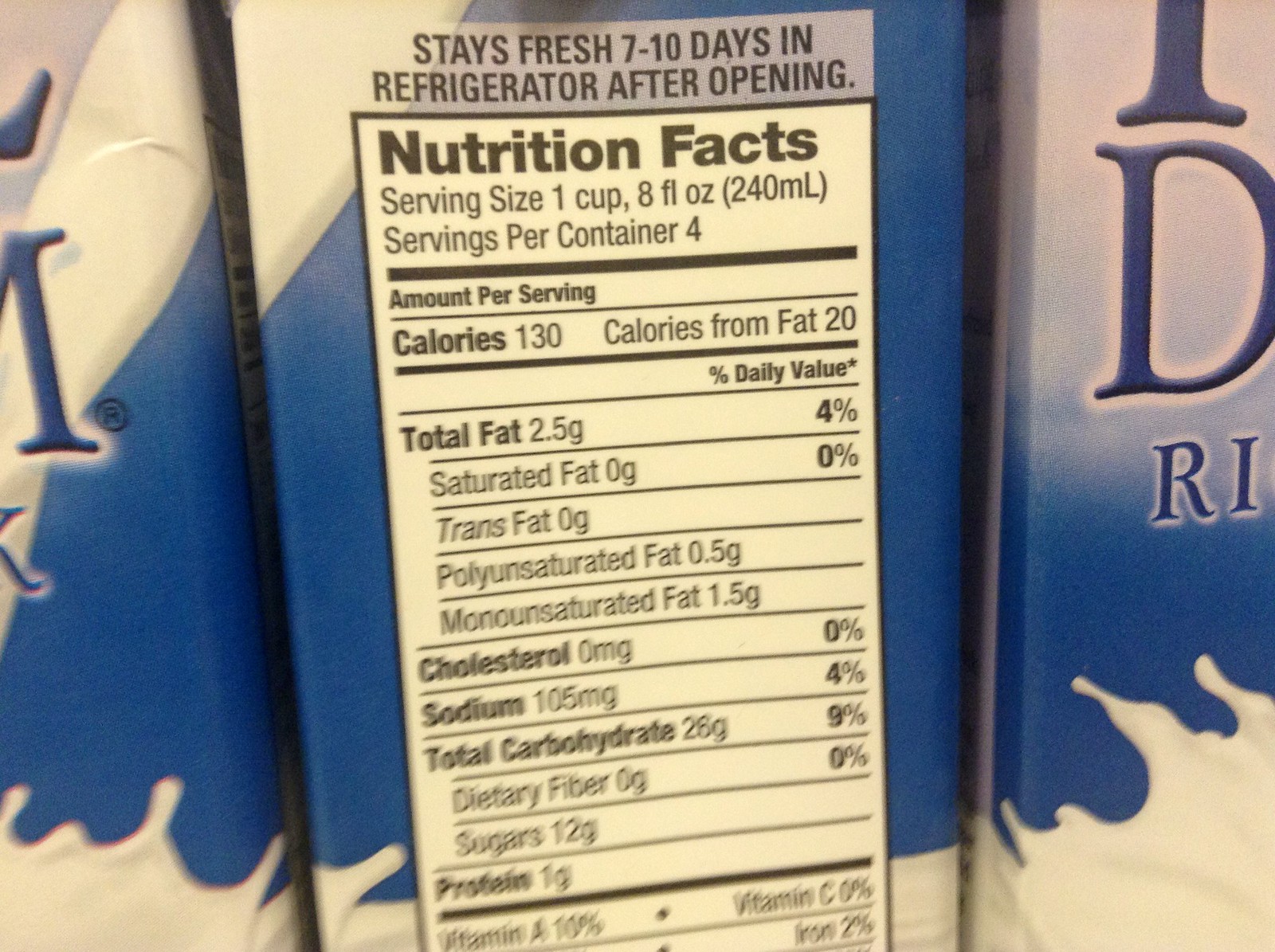This is a photograph of the Nutrition Facts label on a carton of Rice Dream rice milk. The photo features three cartons positioned horizontally, with the center carton displaying the Nutrition Facts label. The cartons are primarily blue, adorned with white imagery of milk splashing at the bottom. The label is primarily dark blue text on a white background. At the top of the label, in capital black letters, is a note: "STAYS FRESH 7-10 DAYS IN REFRIGERATOR AFTER OPENING." Below this is the Nutrition Facts section, detailed in bold at the top. The serving size is listed as one cup (8 fluid ounces, 240 milliliters) with four servings per container. Amount per serving is specified with 130 calories, including 20 calories from fat. The label continues with daily values and nutrients in descending order: Total Fat 2.5 grams (4% DV), with subdivisions for Saturated Fat (0 grams, 0% DV), Trans Fat (0 grams), Polyunsaturated Fat (0.5 grams), and Monounsaturated Fat (1.5 grams). Cholesterol is 0 milligrams (0% DV), Sodium 105 milligrams (4% DV), Total Carbohydrates 26 grams (9% DV), Dietary Fiber 0 grams (0% DV), Sugars 12 grams, and Protein 1 gram. The label also includes daily values for Vitamin A (10%) and Vitamin C (0%), and Iron (2%). The text becomes progressively blurrier towards the bottom, particularly from Saturated Fat downward. On the right side, part of the brand name, "DREAM", is partially visible with a white highlighted capital "D" and "RI" below it. On the left, the letters "M" and "K" are discernible, indicating the partial front of the product label.